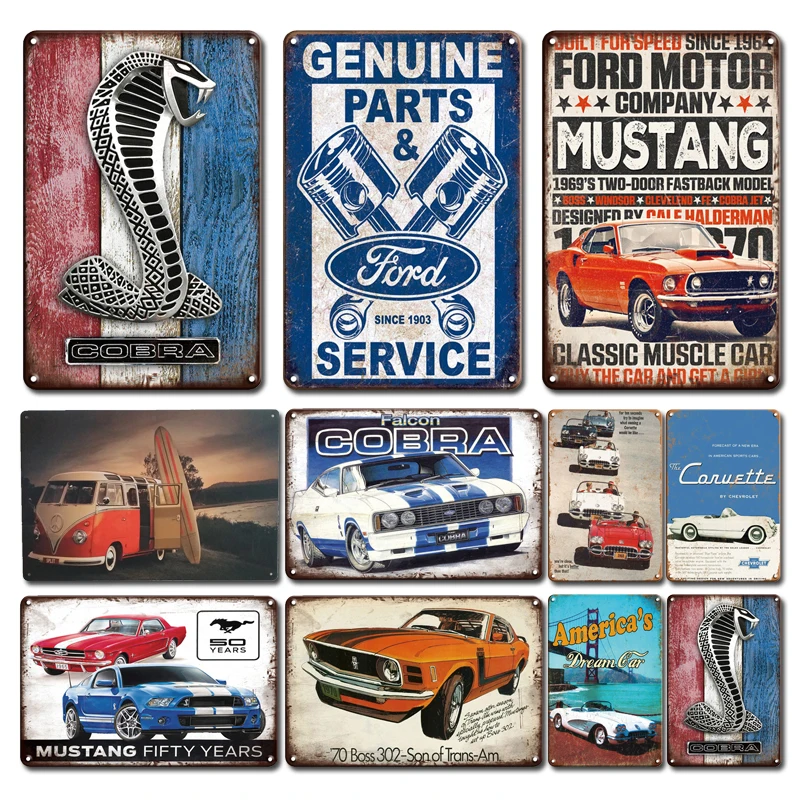This image showcases a vibrant collection of vintage metal signs, each depicting classic car advertisements. Starting from the top left, the first sign features a red, white, and blue background with a silver Cobra emblem in the middle, underneath which "Cobra" is written in black. The top middle sign reads "Ford Genuine Parts and Service" in bold blue and white colors. To its right, another Ford sign displays a classic muscle car with the word "Mustang" prominently in large white letters. 

In the middle row, the left sign portrays a nostalgic Volkswagen van with a surfboard by the water. Centrally, there's a sign featuring the text "Falcon Cobra" in bold lettering. Adjacent to it on the right, a sign displays the iconic Corvette, with the phrase "America's Dream Car" beneath it. 

The bottom row starts on the left with a celebration of 50 years of the Mustang, showcasing two cars, a blue Mustang and a red older version of the Mustang. The middle picture features a large, orange Trans Am labeled "70 base 302 Son of a Trans Am." Finally, reappearing in the bottom right is the Cobra sign, identical to the one at the top left.

Together, these signs create a colorful and nostalgic tribute to classic muscle cars, predominantly featuring Ford Mustangs and Cobras, with accents of other iconic vehicles like the Volkswagen van and Corvette.